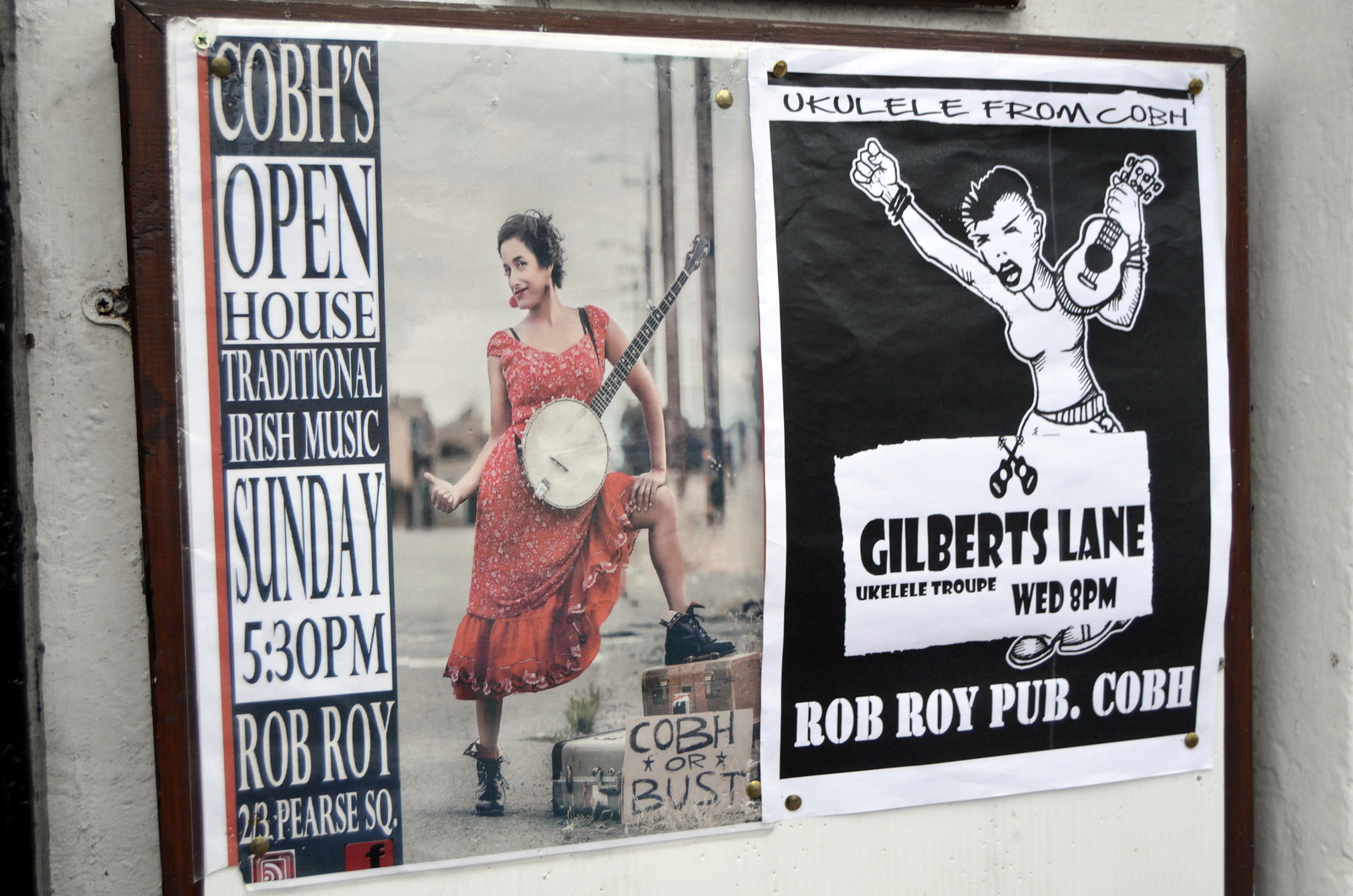This photograph captures two distinct posters affixed to a white board mounted on a white wall, potentially positioned along a city street. The left poster prominently features a woman in a vibrant red dress, striking a hitchhiker pose with a banjo in hand and her leg resting on a piece of luggage. She exudes a playful energy, indicated by her thumbs-up gesture. The accompanying text reads: "Cobb's Open House, Traditional Irish Music, Sunday, 5.30pm, Rob Roy, 2-3 Prius Square." 

Conversely, the right poster is a striking black-and-white illustration of a woman with a mohawk haircut, energetically holding a ukulele in her left hand while appearing to be mid-yell. The text on this poster announces: "Ukulele from Cobb, Gilbert's Lane, Ukulele Troupe, Wednesday, 8pm, Rob Roy Pub." The diverse color palette of red, tan, black, white, and gray adds to the visual interest of the posters, which advertise musical performances at the Rob Roy Pub in Cobb. The angled shot suggests the photo was taken candidly, although it's unclear whether it was indoors or outdoors, or during day or night.